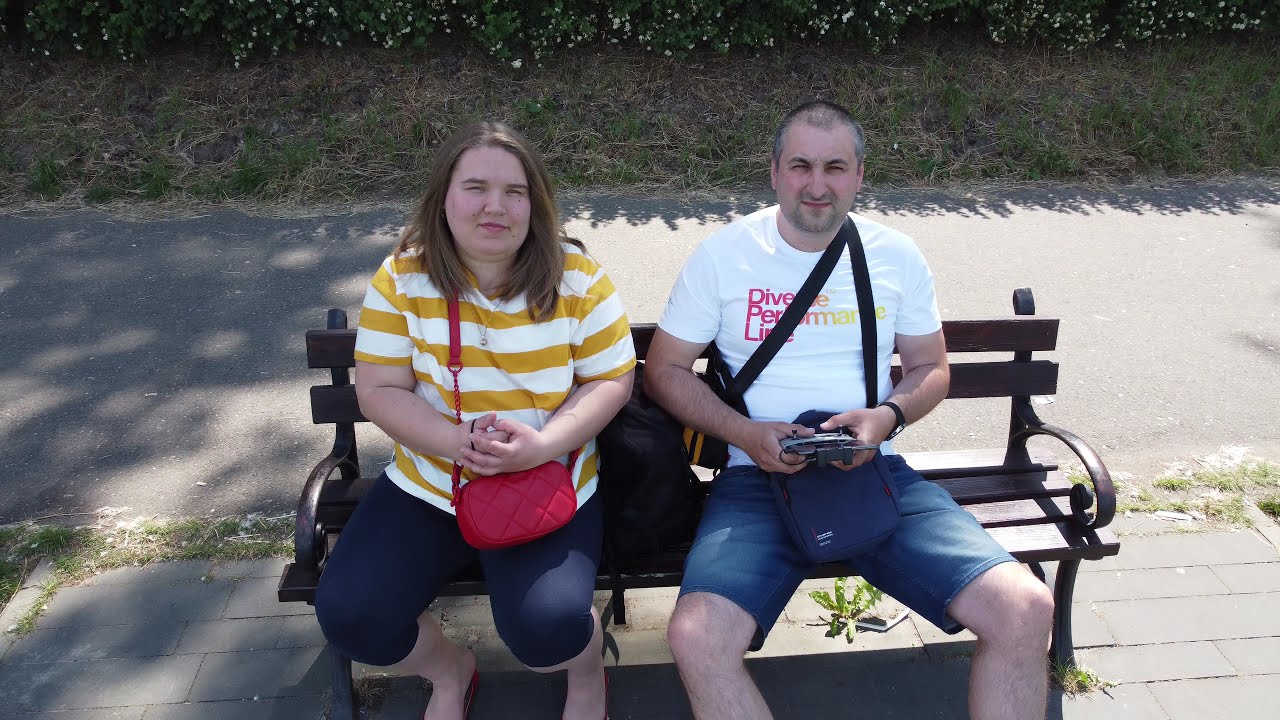In this photograph, there are two individuals, a man and a woman, seated on a park bench facing the camera. The man on the right is holding what appears to be a drone controller, suggesting he may be operating the drone that's capturing the image. Both individuals are overweight; the woman on the left is noticeably so, possibly by around 100 pounds. She has straight, shoulder-length hair and is wearing a cotton, orange and white striped shirt paired with blue jean capris. A pillowy red purse is draped across her body. She sports pink lipstick and, like the man, squints at the camera with a neutral expression. The man is balding, dressed in a white T-shirt with partially obscured text, "Dive, Pear, and Maine Live," due to a crossbody camera case strap. He is also wearing denim shorts. The backdrop features a narrow road flanked by flower bushes and shrubs, contributing to the park-like setting.